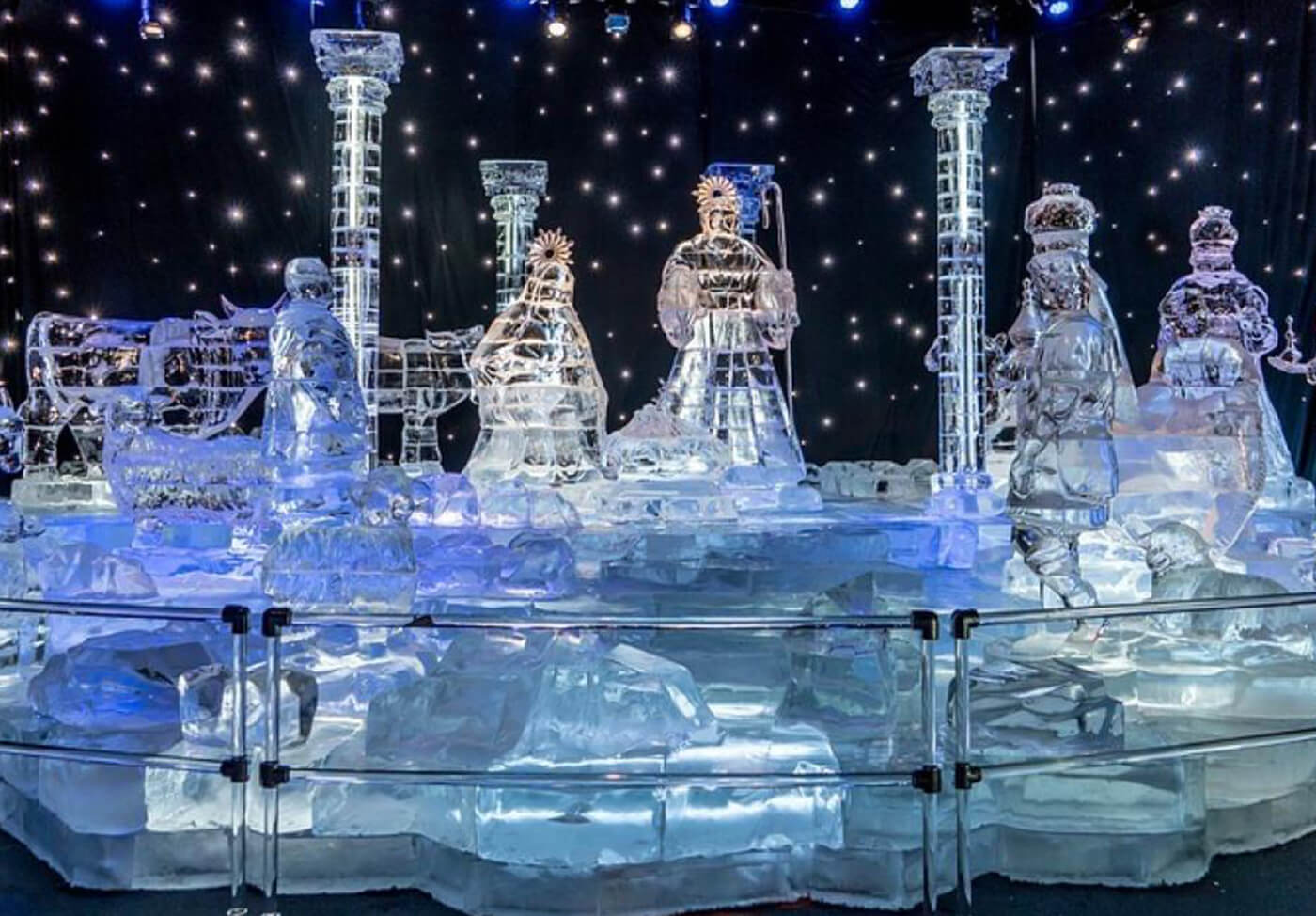This intricately detailed photograph captures a scene of a meticulously crafted ice sculpture nativity set, enclosed within a circular metal or plexiglass railing. It depicts several glass-like figurines resembling characters from the nativity story—Mary, Joseph, the three wise men wearing crowns, and various farm animals. Positioned centrally, there appears to be an ice cradle symbolizing the birthplace of baby Jesus, although the baby itself is not distinctly visible. The scene is enriched by scattered ice blocks and formations depicting the surrounding terrain, creating an immersive setting. Above the nativity, the background is meticulously illuminated with countless bright white dots mimicking a starry night sky, adding a magical touch to the entire composition. The thoughtful arrangement and unique use of lighting make this ice sculpture ensemble a captivating piece of art.